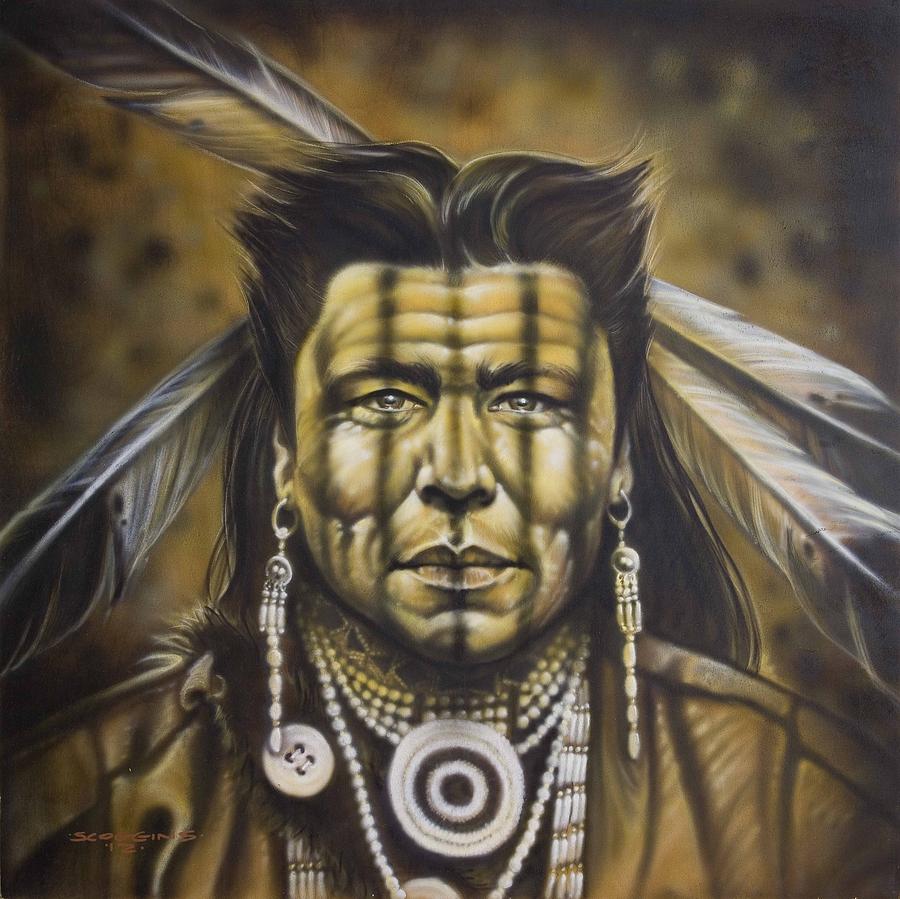The image depicts a close-up illustration of a Native American man with distinctive facial features and adornments. He has a combination of short, spiky hair on top and longer hair in the back, adorned with four large white feathers tipped in black. Two feathers on the left side point upwards and sideways, while two on the right side point downward and are positioned above his ear. His complexion appears to be covered in a yellowish-orange paint with five prominent vertical black stripes running down his face from the forehead to his jawline, one of which goes through each eyebrow and another down the center of his face. His expression is serious and somewhat somber, with no discernable smile.

He is wearing long dangly earrings and multiple pearl or beaded necklaces with rings and buttons around his neck. His clothing consists of a caramel or tan-colored shirt or jacket that can be seen up to his shoulders and chest but not his arms. The background is blurred and features brownish tones, giving the impression of being in low light or shadow. The overall color scheme of the image includes shades of brown, yellow, and white, contributing to a warm, earthy aesthetic.